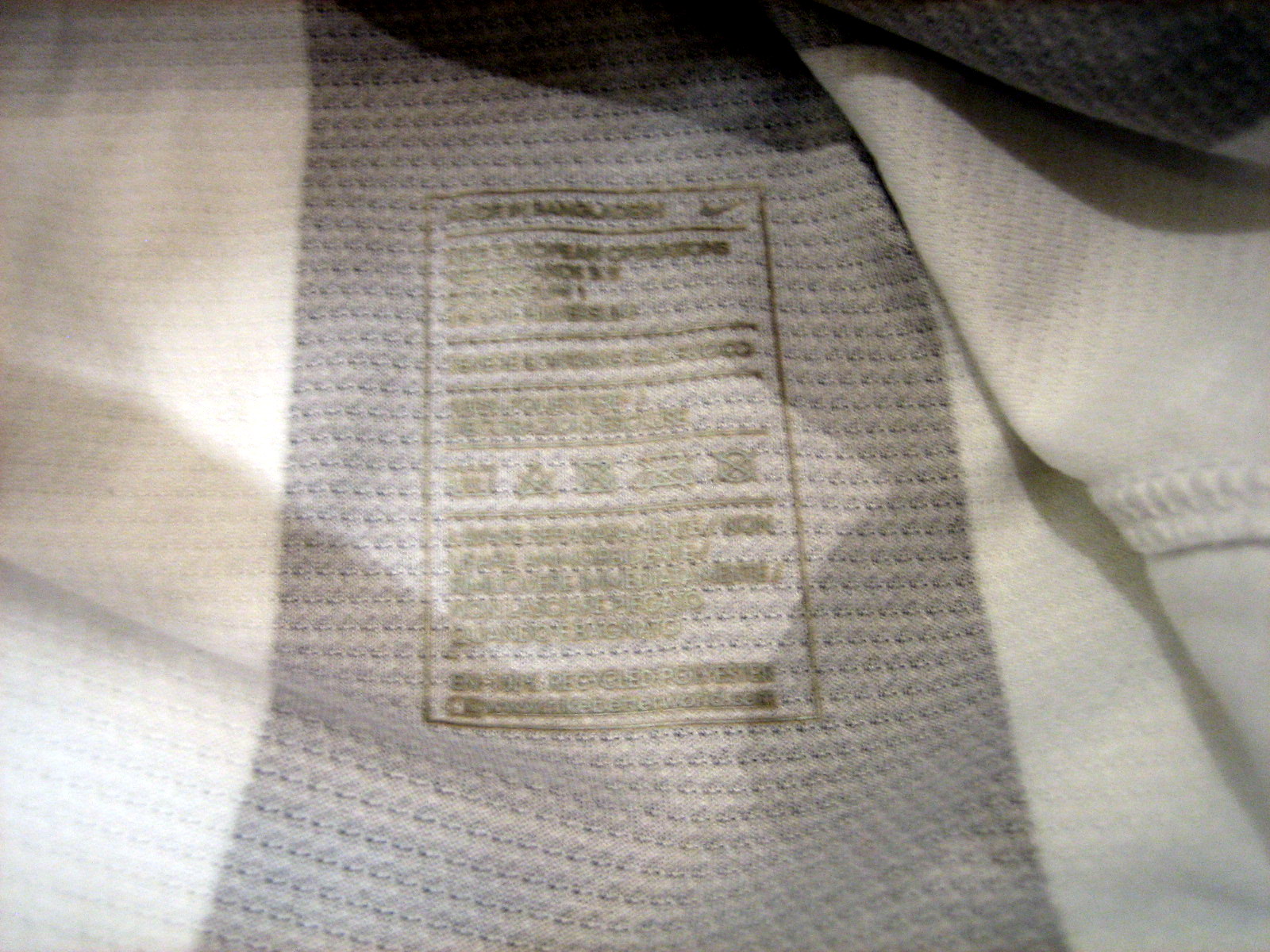The image is a detailed close-up photograph of a white fabric with visible folds and a textured surface. At the center of the fabric, a large, grayish rectangle appears, which seems to be the tag of a garment. The tag is partially obscured by sunlight but features the Nike swoosh logo and golden writing that reads "Bangladesh," indicating its place of manufacture. Although the rest of the text on the tag is out of focus, the high quality of the fabric is evident. The material, possibly cotton, showcases its fine craftsmanship through the visible creases and overall pristine condition.